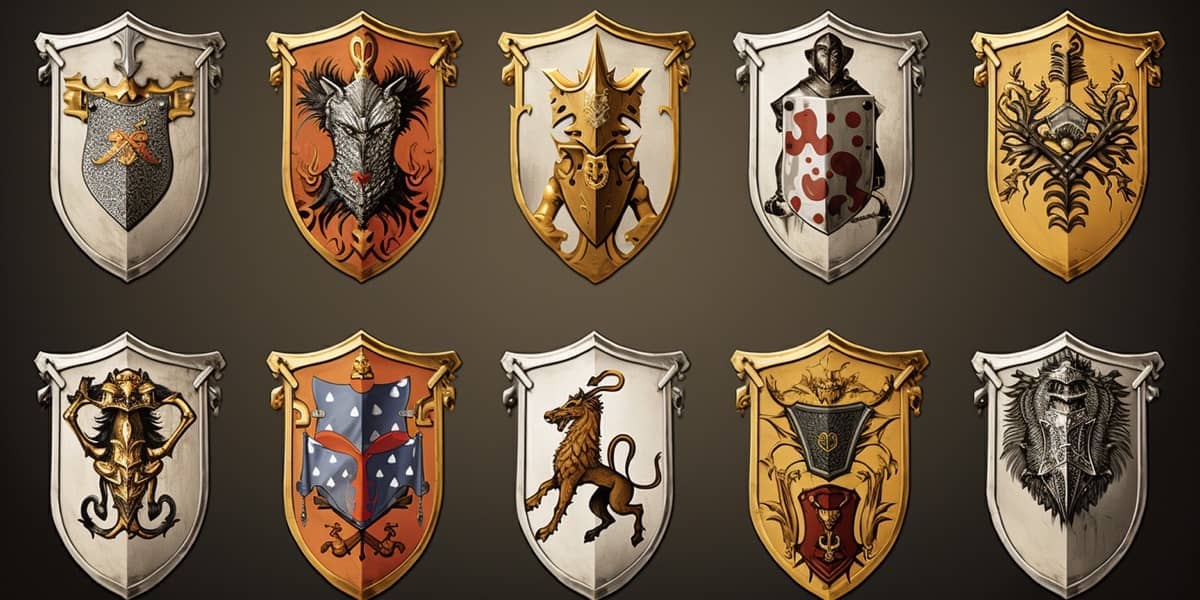This detailed, colour image shows ten heraldic shields arranged horizontally in two rows of five, set against a dark greyish-brown background. Each shield displays unique icons, ranging from animals to mythological and knightly symbols, all in a muted color palette of greys, oranges, whites, yellows, and golds. In the top row, the first shield is white with a smaller grey shield detailed in gold, followed by an orange shield featuring a grey figure, and a white shield edged in gold with a golden icon. Next is a silver shield with a grey humanoid figure holding a white and red shield, and finally a gold shield with a brass, twisted, spider-like decoration. The bottom row begins with a silver shield with gold detailing, followed by an orange shield with blue miniatures and white dots. The next shield is silver with a mythological horse-like figure in brown, flanked by a gold shield with intricate grey and brown patterns, and ends with a silver shield sporting a silver emblem. The shields are uniformly shaped, presenting a medieval aesthetic and showcasing a variety of symbols such as shields, knights, animals, and even a scorpion-like creature, each emblematically representing different families or knighthoods.